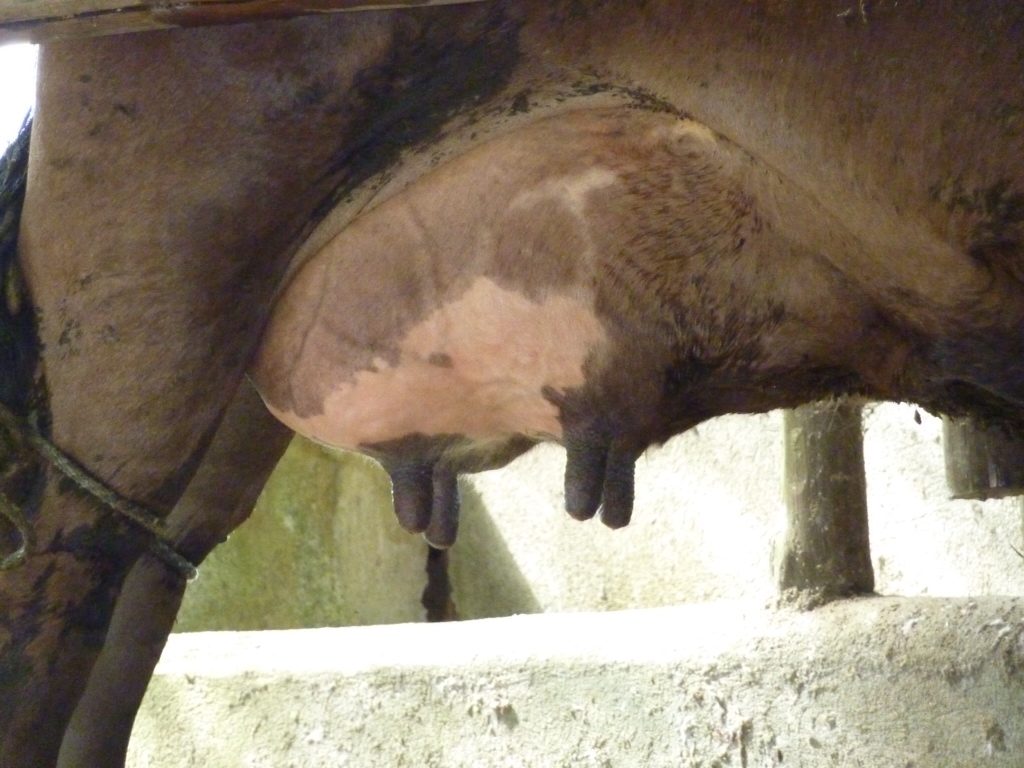The photograph is a close-up shot focusing primarily on a cow's udders and the underside of its belly. The cow's body is a mixture of dark brown and black, and the skin appears stretched, suggesting potential pregnancy. The four visible udders are black and engorged, protruding from a pink underbelly, which gives a painful appearance. The cow's hind legs are bound together with a black rope, adding to the distressing nature of the scene. The background reveals a dirty room with gray speckles on what appears to be a white stone or concrete wall, contributing to the overall depressing and somber setting. The image is clear, enhanced by natural daylight, emphasizing the stark details.